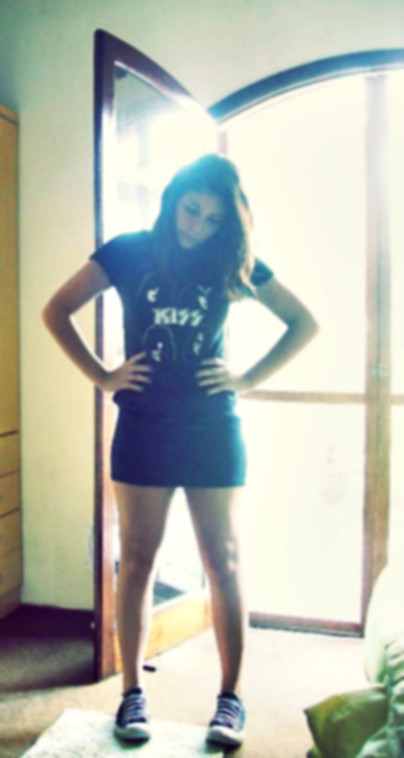The image portrays a teenage girl standing confidently in front of an open wooden door with a glass middle, through which sunlight is pouring in, casting a bright and overexposed glow over the scene. The bright sunlight highlights a slightly blurred and grainy quality to the photo. She is facing the camera with her hands firmly on her hips, and her head slightly angled downward, suggesting a self-assured stance. 

The girl is dressed in a short-sleeved black t-shirt displaying the KISS logo prominently in white, accompanied by faint images of the four band members' faces. Her long, dark brown hair cascades over her shoulders, partially obscuring the t-shirt's design. She pairs the t-shirt with black shorts that fit snugly around her upper thighs. On her feet, she sports blue and white sneakers with distinct purple and blue shoelaces, adding a touch of color to her monochrome outfit. 

The setting appears to be indoors with a white or potentially yellow wall due to the lighting, and a light brown door adorned with a screen that is barely discernible due to the intense sunlight. The girl stands on a beige floor covered by a white rug, with some green object, possibly clothing, visible in the bottom right corner. Additionally, a brown armoire stands against the wall, contributing to the room's decor. The photograph captures a moment of youthful defiance and style, radiating through the highlighted and overexposed composition.